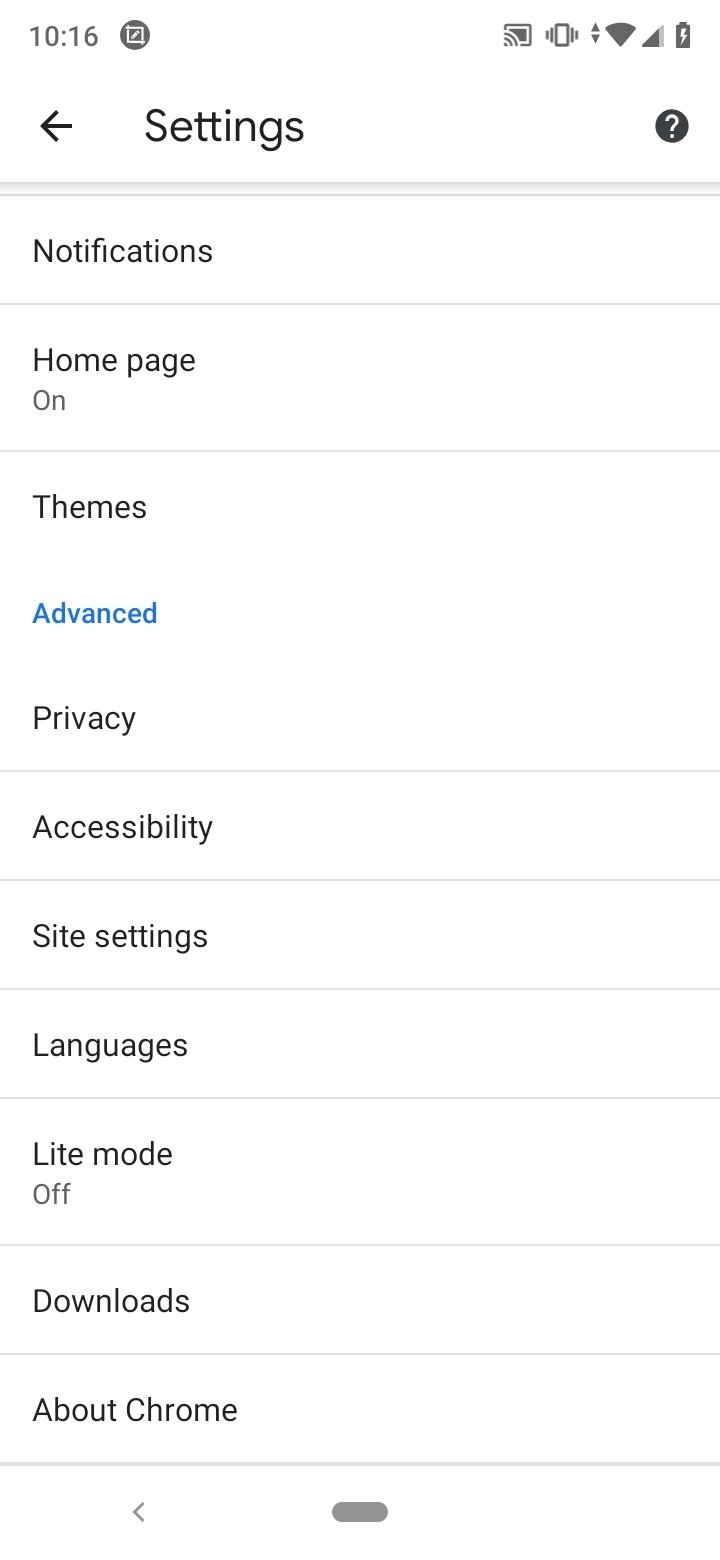This is a detailed screenshot of a settings screen, likely from a phone or tablet. The background is white, and most of the text is gray, aligned towards the left. At the top, the heading "Settings" is prominently displayed in black, with a faint blue underline. To the far right of the heading, there is a black circle with a question mark, suggesting it is clickable for additional information or help.

The list of settings options is displayed in a left-aligned column:

1. **Notifications** - Status: ON (Gray text)
2. **Home Page** - (Gray text)
3. **Themes** - (Gray text)
4. **Advanced** - (Blue text)
5. **Privacy** - (Gray text)
6. **Accessibility** - (Gray text, separated by a faint blue line)
7. **Site Settings** - (Gray text, separated by a faint blue line)
8. **Languages** - (Gray text, separated by a faint blue line)
9. **Light Mode** - Status: OFF (Gray text, separated by a faint blue line)
10. **Downloads** - (Gray text, separated by a faint blue line)
11. **About Chrome** - (Gray text, separated by a faint blue line)

Each section is delineated by faint blue lines, adding a subtle structure to the settings list.